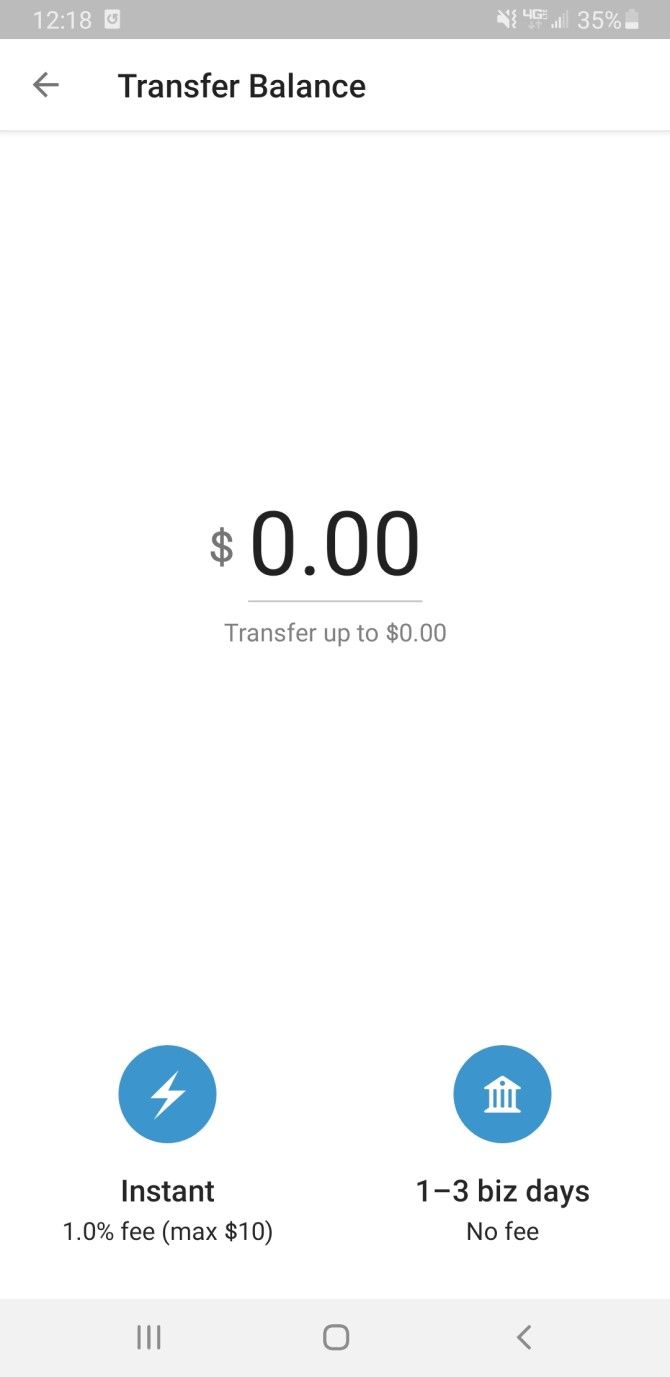The image displayed on an iPhone screen reveals a banking app interface, showing a partial balance transfer screen. The phone’s battery level is at 35%, with a moderate connection signal. The time displayed is 2:18. At the top of the screen, the title "Transfer Balance" is prominently presented in black letters alongside a left-facing gray arrow. Directly below, a thin gray line segments the screen. The mostly blank white background suggests little content has been input.

In the center of the screen, the amount "0.00" is shown, indicating no balance has been entered for transfer yet. It instructs the user that they can transfer up to "0.00." Beneath this, there are two options for making the transfer: one providing an "Instant" transfer with a 1.0% fee, capped at a maximum of $10, and the second offering a transfer within "1-3 business days" with no fee. These options are highlighted in blue circles.

At the bottom, a gray navigation bar includes three vertical lines on the left, likely representing a menu, and a gray home button in the center. Another gray arrow points to the left, suggesting a back function.